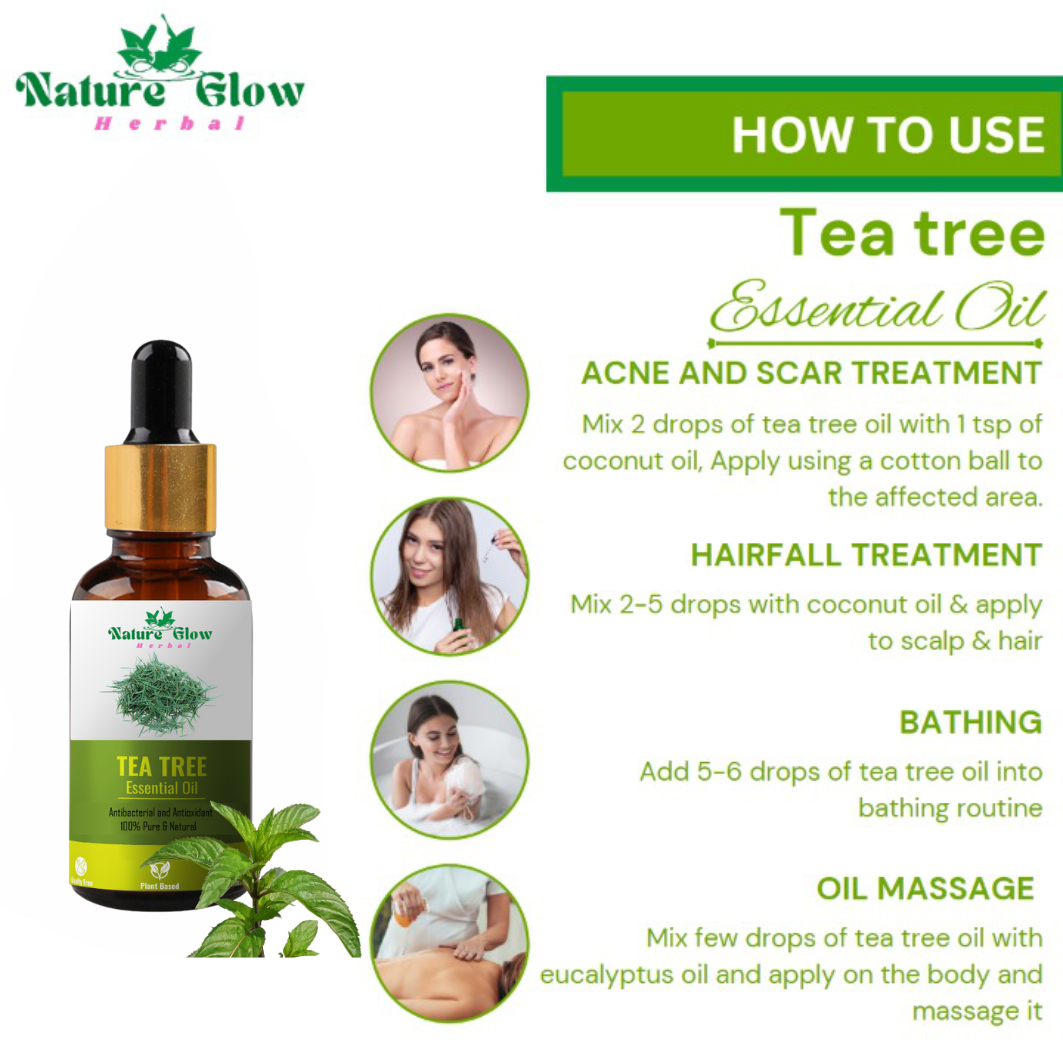The image is an advertisement or instructional guide for "Nature Glow Herbal" tea tree essential oil, set against a white background with predominantly green text. In the upper left-hand corner, the logo "Natural Nature Glow Herbal" is displayed. A large headline reads "How to Use" followed by "Tea Tree Essential Oil." The guide outlines several applications: for acne and scar treatment, it suggests mixing two drops of tea tree oil with one teaspoon of coconut oil and applying it with a cotton ball; for hair fall treatment, it advises mixing two to five drops with coconut oil and applying to the scalp and hair. For bathing, users should add five to six drops into their bathwater, and for an oil massage, mix a few drops with eucalyptus oil and massage onto the body. These instructions are visually supported by circular images depicting a woman applying the oil on her face, hair, in a bath, and during a massage. The product itself, a bottle with a dropper top, is positioned to the left, emphasizing its easy application method.